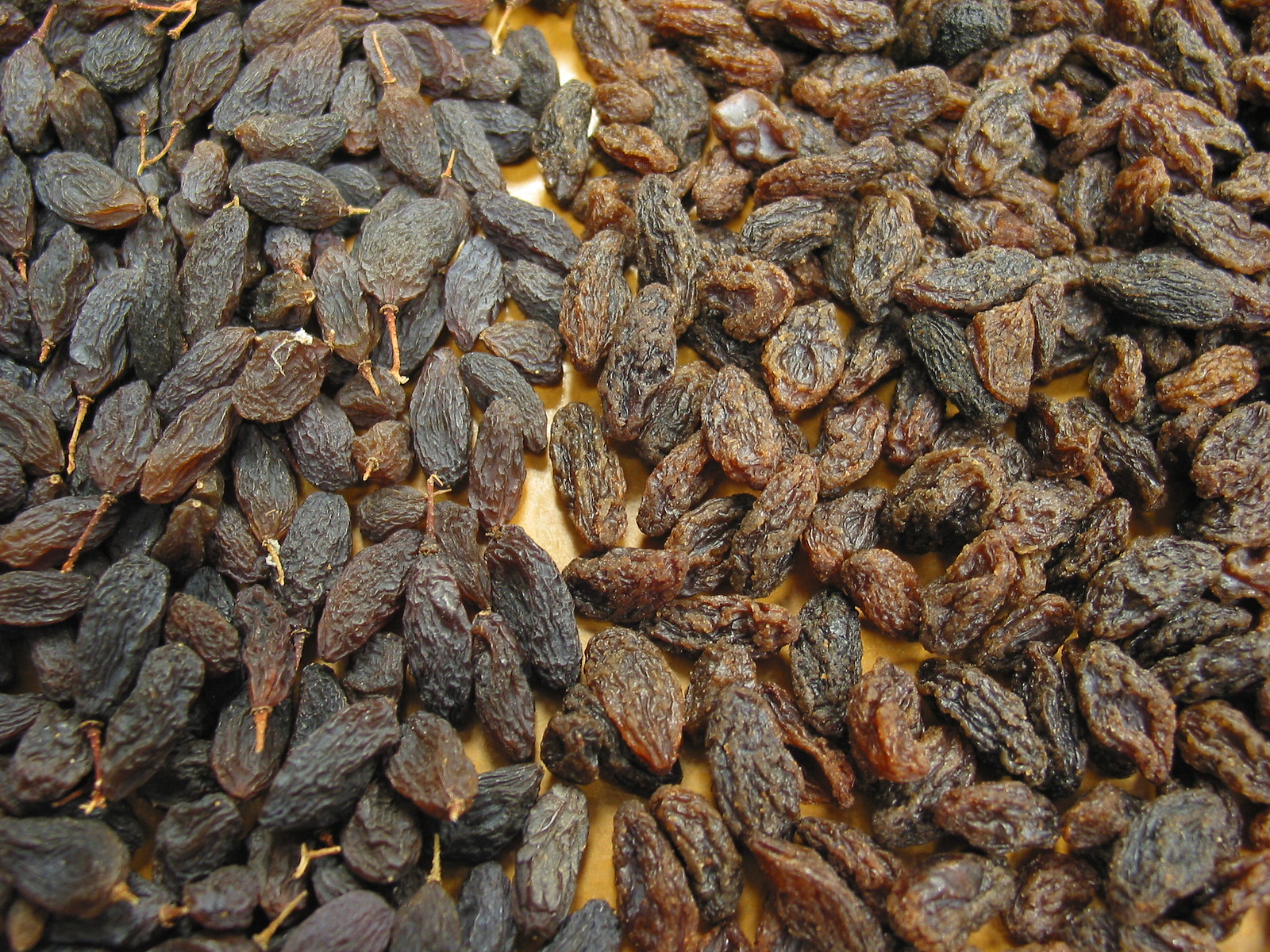This is an overhead color photograph featuring a large quantity of dried raisins arranged on a light tan wooden table. The image prominently displays these dark brownish-blackish and lighter brown raisins in a close-up view, revealing intricate details of their texture. To the left side of the photograph, the darker raisins are distinctly visible with their stems intact, giving them a slightly rugged appearance. Conversely, the raisins on the right appear lighter in color and lack visible stems, suggesting a possible difference in processing or aging. The raisins are heaped together, potentially numbering in the hundreds, and there's a subtle yellow hue peeking through from underneath, possibly from the surface they are placed on. Notably, there are no people, date stamps, or text within the image, allowing the viewer's attention to focus solely on the varying shades and forms of the dried fruit.